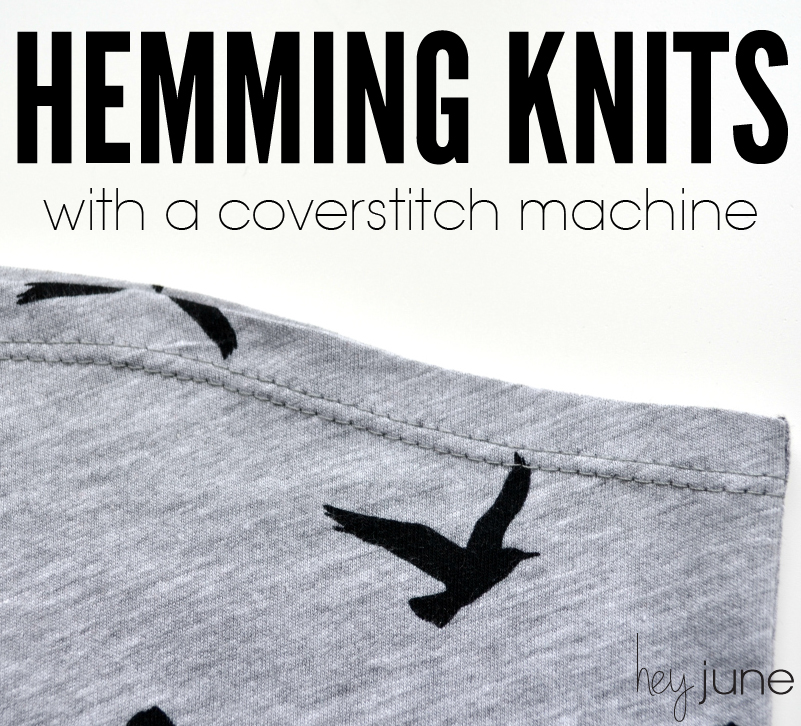The image appears to be an advertisement or instructional cover for "Hey June" entitled "Hemming Knits with a Coverstitch Machine." The title is prominently displayed at the top in bold, tall capital letters, "Hemming Knits," followed by a smaller, lowercase, Century Gothic font stating "with a coverstitch machine." The image is in grayscale, featuring a close-up of a heather gray fabric, likely a t-shirt sleeve, that has been hemmed using a cover stitch machine. The sleeve showcases the double stitch technique along the edge. The fabric also features a black outline pattern of seagulls in flight, with one whole silhouette visible and others partially cut off. A watermark in the bottom right corner reads "Hey June" in a script font. The overall composition suggests that this is a detailed guide or tutorial on how to hem knits effectively using a cover stitch machine, likely including step-by-step instructions, techniques, and common mistakes to avoid.